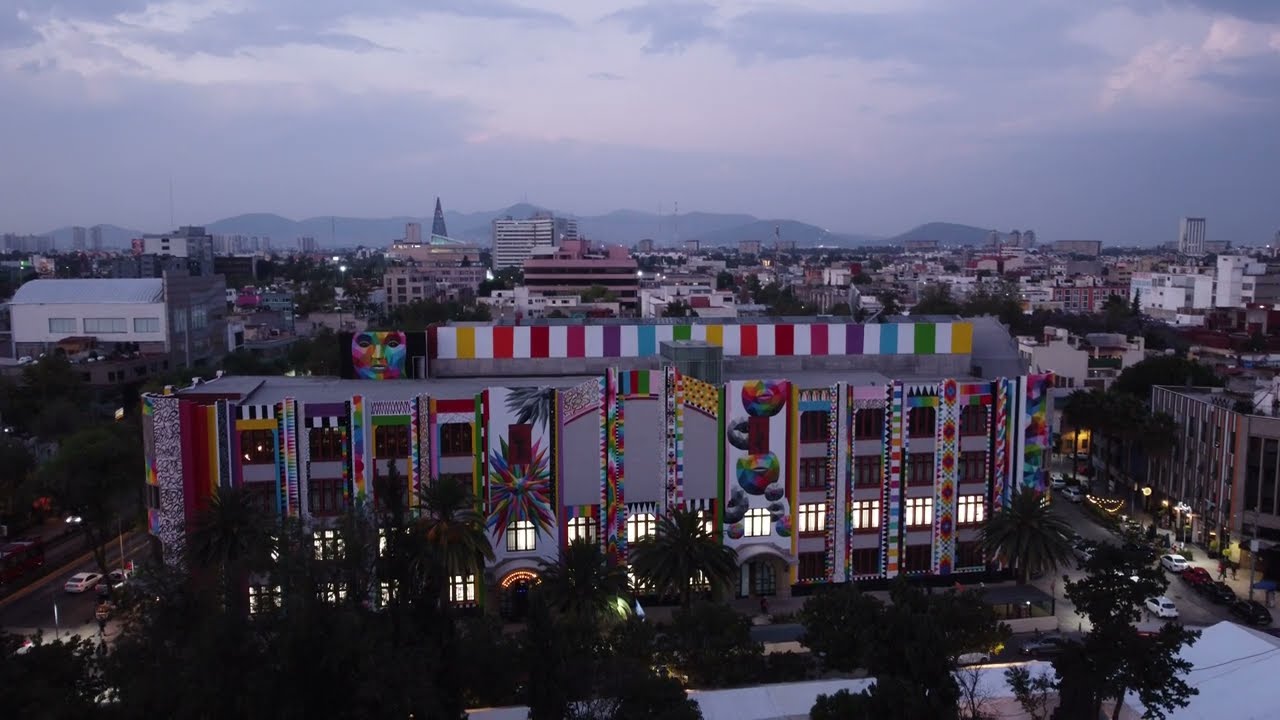The image presents an aerial view of a sprawling metropolis under a mostly gray, cloud-filled sky, likely captured during the evening hours. The focal point of the image is a distinctive concrete building in the foreground, approximately four or five stories tall, adorned with a vibrant rainbow stripe against a primarily off-white backdrop. The building features multiple artistic renderings resembling 3D facial art, with window frames in a dark red hue. Surrounding this colorful structure are numerous buildings, outlined in red and white, interspersed with abundant trees filling every possible space. The city's layout is visible with streets and light poles threading between the buildings. In the far distance, a mountain range can be seen through the fog, adding to the scene’s depth and sense of scale.